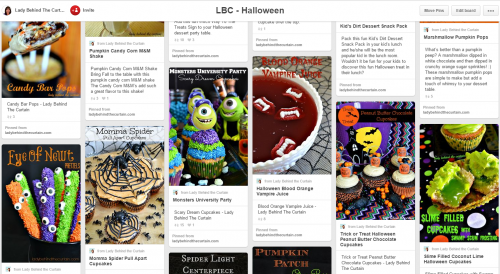This screenshot captures a detailed view of a Pinterest board titled "LBC Halloween," curated by Lady Behind the Curtain. The board is a rich collection of Halloween-themed baking ideas, featuring an array of creative desserts like cupcakes, cookies, and other sweet treats. 

In the top left corner, an avatar of Lady Behind the Curtain is prominently displayed. To the right of this image, you'll find a red "Pinterest Add" button and an "Invite" button, allowing for easy sharing and collaboration. The board’s title, "LBC Halloween," is clearly visible, and on the far right side of the screen are the "Move Pins" and "Edit Board" buttons, providing organizational options.

The content is vibrant and varied, starting with candy bar pops, and moving into a pumpkin candy corn M&M shake. Near the center of the board, visually striking Monster University Party Cupcakes catch the eye. To their right is a spooky Blood Orange Vampire Juice. Further right is a particularly ghoulish treat, Slime Filled Cupcakes with Swamp Scum Frosting, featuring green frosting and eerie green filling.

This board is a treasure trove of inspiration for anyone looking to add a creative twist to their Halloween festivities.